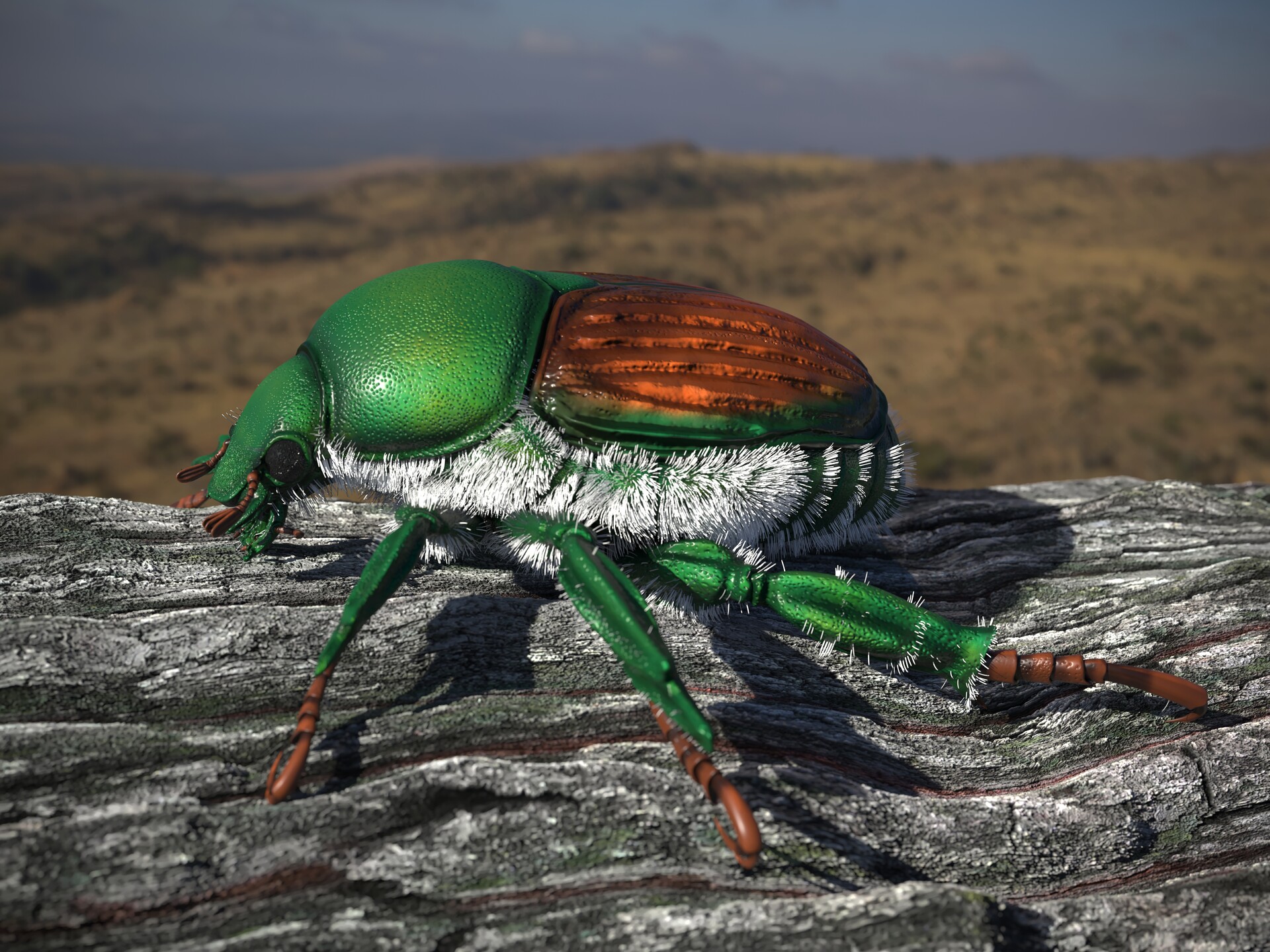This highly detailed, photorealistic image captures a close-up of a vibrant beetle perched atop weathered, grayish wood that shows traces of lichen growth. The beetle, likely a type of Japanese beetle, is facing to the left and stands out vividly against the blurred backdrop of a grassy field and a cloudy sky. Its head and upper body are a striking emerald green, while its rear wing plates and antennae shimmer with a metallic bronze-copper hue. The beetle's legs, three of which are visible extending from its body, are bright green adorned with sparse white hairs, and end in brown tips. Its underbelly is covered in fuzzy, grayish-white hair, adding to its detailed texture. The background of the image features a desolate, shrub-laden landscape with hints of sagebrush against a gray, cloud-filled sky, all carefully blurred to draw attention to the intricate details of the beetle, which dominates the frame.